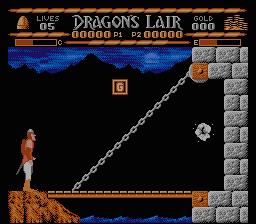In this image from the video game "Dragon's Lair," the title is prominently displayed at the top in grey lettering. To its left, there is an indicator showing that the player character has 5 lives remaining. On the opposite side, to the right, is a symbol representing gold, currently at a value of 0. Below this, a health bar is visible, indicating that the player’s health is about halfway depleted. The scene at the bottom of the screen depicts the character traversing a drawbridge. Additionally, there is a square icon with the letter "G" situated at the top right corner, just above the drawbridge, suggesting an in-game element or objective related to the scene.